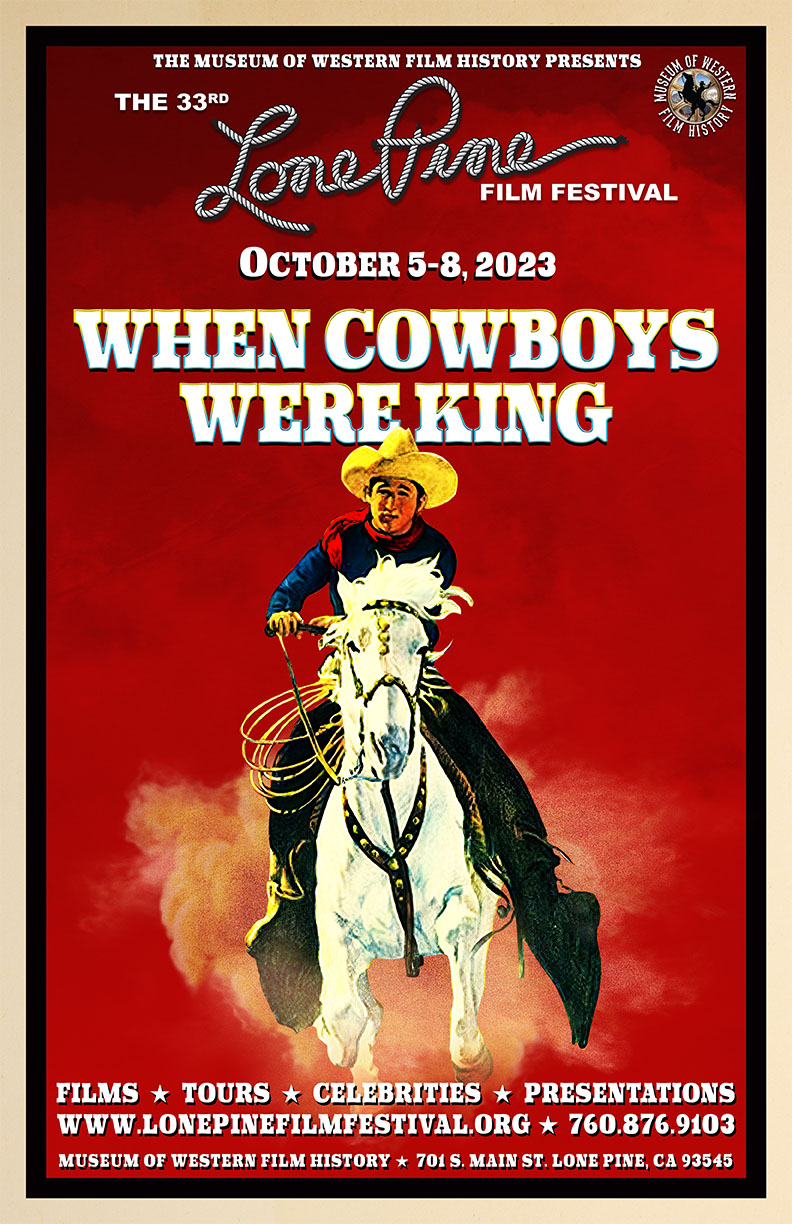The poster, dominated by a solid red background, announces the Museum of Western Film History's presentation of the 33rd Lone Pine Film Festival, held from October 5th to the 8th, 2023, with the tagline "When Cowboys Were King." At the center, a detailed portrait depicts a cowboy riding a galloping white horse, both facing forward. The cowboy is authentically outfitted with a yellow cowboy hat, a red scarf, a blue shirt, black pants, and likely black boots, which blend into the horse's body. He clutches the reins of the horse, which sports a black leather bridle with gold accents. Additionally, a rope rests on the cowboy’s hip. Below the image, the poster highlights "Films, Tours, Celebrities, Presentations" and provides a website (www.lonepinefilmfestival.org) and contact details (760-876-9103, 701 Main Street, Lone Pine, California 93545) for further information.